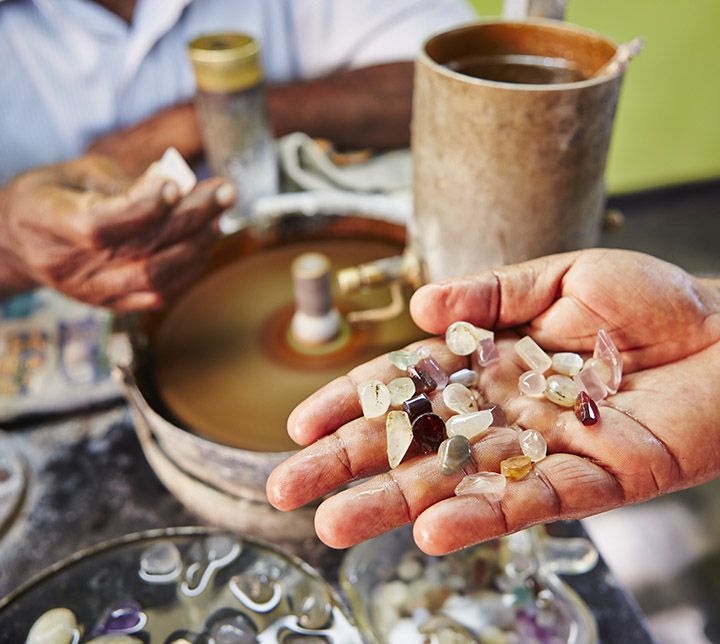The photograph showcases a worn, wrinkled hand holding an assortment of polished rocks in an open palm. The hand features various stones including a pink diamond-shaped rock, a white rectangular rock, a white oval-shaped rock, and numerous others of different colors such as black, gray, orange, red, violet, amber, and green. In the background, a grinding wheel encased in a tannish bronze-colored bowl is in motion, connected to a water-filled cylinder with pipes and tubes, suggesting a rock-tumbling or polishing apparatus. The top left corner of the image reveals another person, slightly out of focus, wearing a blue button-up shirt with the top button undone, holding a large white rock. The bottom left corner contains various bowls filled with water-soaked rocks, waiting to be worked on. The scene is set against a dirty gray surface, depicting a workspace dedicated to the meticulous process of rock polishing.